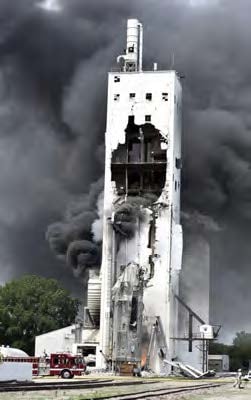In this image, a tall, narrow, rectangular building is experiencing a devastating incident, likely an explosion or fire, given the massive black smoke billowing into the sky, obscuring much of the background. The building, which resembles a high-rise or large industrial structure, has a significant hole on its side and shows damage near the top where the wall appears caved-in, forming a mouth-like shape. A crack runs from the damaged area down the building, resembling a fracture. At the base, material is spilling out towards the viewer. 

A red firetruck is visible at the bottom left, along with some people seemingly evacuating the scene. The foreground reveals a strip of sidewalk or road, and there are hints of green grass and trees scattered along the horizon. Train tracks appear to lead to and around the building, suggesting an industrial or agricultural setting. The overall color of the image is dominated by grayish-black tones from the smoke, with the only notable colors being the red firetruck and some green foliage. The scene is framed in portrait orientation, emphasizing the towering presence of the smoke-engulfed structure.